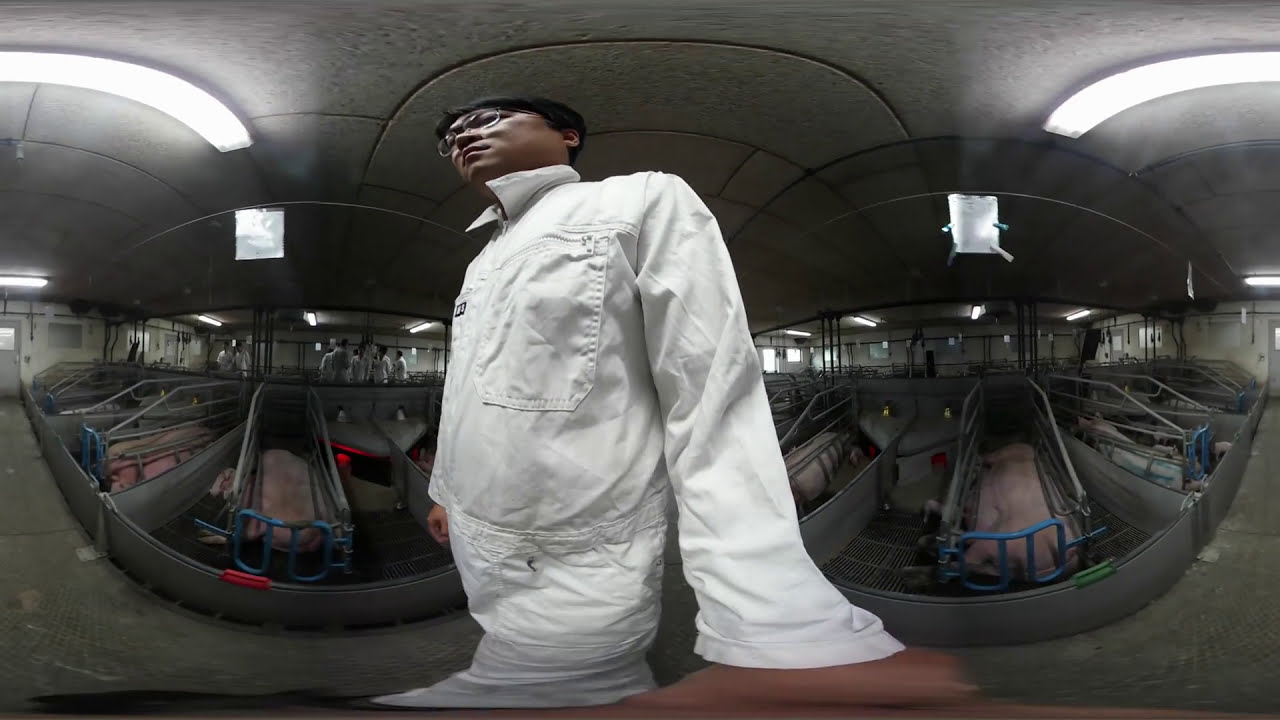In this fisheye lens photograph, a young Asian man with dark hair and glasses is depicted in an industrial factory or farm setting, wearing a white jumpsuit with long sleeves and a turned-up collar. The image, which appears blurred and distorted, possibly from being taken with a webcam or through a filter, only shows him from the waist up. The background features pens or enclosures that likely hold blurred, indistinct animals, possibly hogs. Further in the distance, other individuals in white outfits can be seen, as well as various lights on the ceiling, including square and curved fluorescent lights. The setting is well-lit, with doors on both the left and right sides. The man might be holding a selfie stick, further contributing to the fisheye perspective’s curvature.